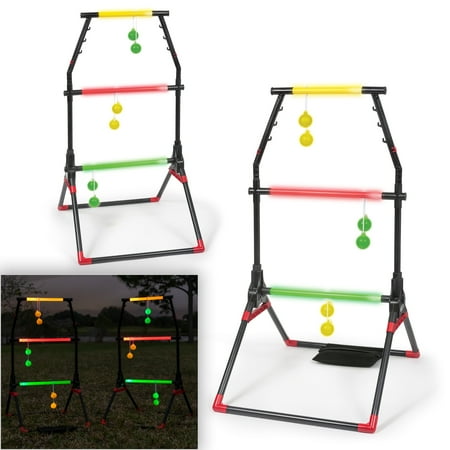The image showcases a vibrant ladder ball game designed for outdoor play, emphasizing its glow-in-the-dark feature. Set against a plain white background, the photo highlights two plastic ladder ball racks, each stabilized by splayed legs. These racks are adorned with three brightly colored horizontal bars: a green bottom bar, a pink middle bar, and a yellow top bar. Weighted balls connected by cords hang from these bars—green balls on the bottom bar, pink or yellow balls on the middle bar, and yellow balls on the top bar. In the lower right corner, an inset photo demonstrates the glow-in-the-dark capability, with the crossbars and balls emitting a bright illumination against a dark, night sky. Additionally, a storage box for the ladder ball racks is depicted in the bottom left corner, underscoring the game's portability and ease of storage.